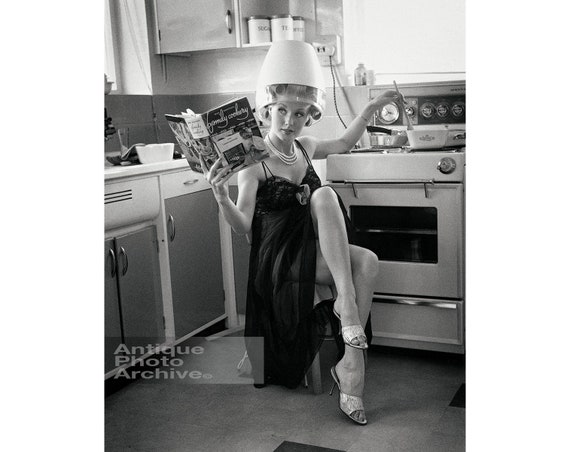This black-and-white photograph, likely from the 1950s or 1960s, captures a vintage domestic scene of a woman multitasking in her retro kitchen. Seated on a stool, she is adorned in a black, satiny negligee and open-toed high-heeled slippers, her legs bare and crossed suggestively. A string of pearls enhances her attire, and her hair is set in curlers beneath a helmet-style cap hair dryer, which is plugged into the wall behind her. With her left hand, she stirs a casserole dish on the kitchen range, while her right hand holds an open cookbook labeled "Family Cooking." The woman gazes slightly off to the left, merging domesticity with a sensuous pose. The kitchen, characterized by its vintage cabinets and countertop, includes visible canisters for sugar, tea, and coffee on a shelf above. The timelessness of the scene is marked by the words "Antique Photo Archive" in the lower left-hand corner of the image.